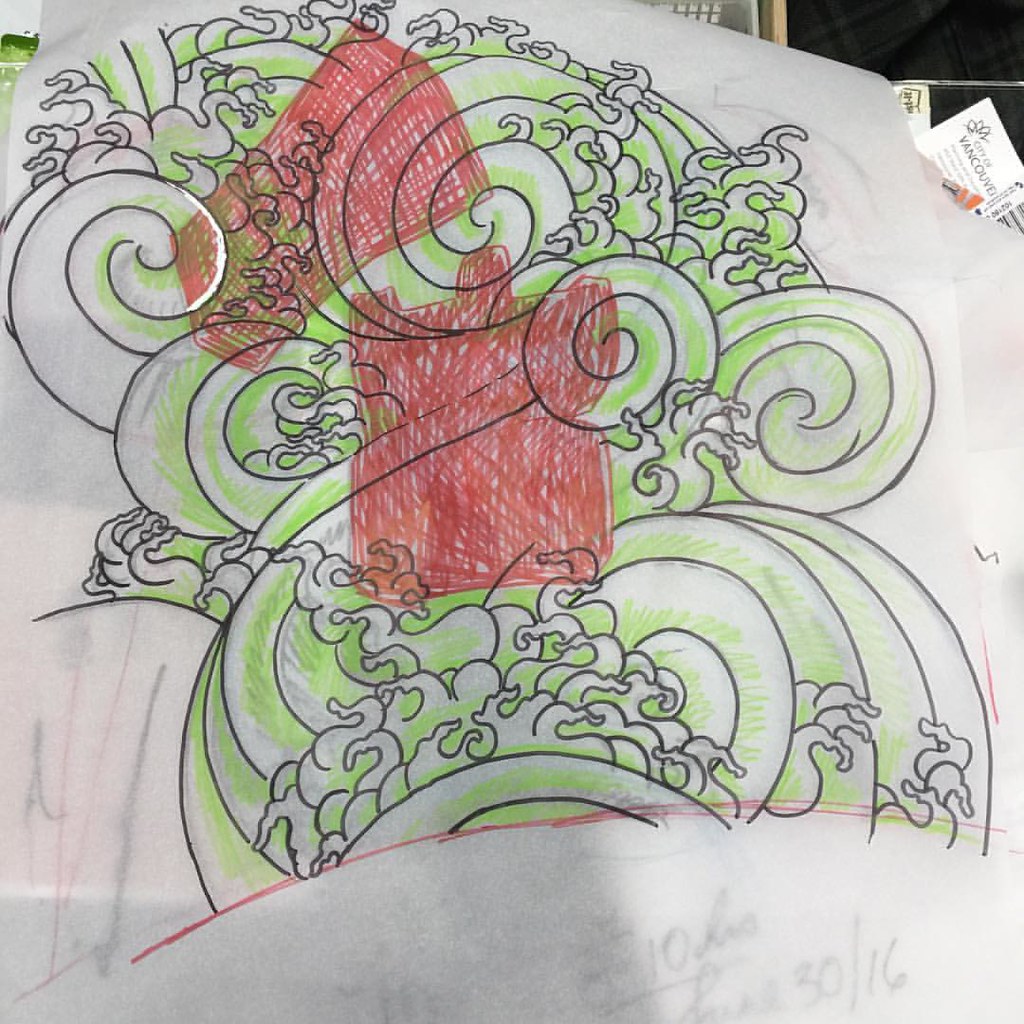A detailed illustration on a white sheet of paper occupies the center of the image, surrounded by a minimalistic background with a notable black corner in the upper right, adjacent to a white piece of paper labeled "City of Vancouver." The primary artwork features a red, curved line at the bottom, from which intricate black linework emerges, resembling waves that eventually transform into more complex, wider-angled circular and spiral patterns. These patterns are predominantly white with delicate touches of lime green shading, giving the design an eclectic yet cohesive feel. Amidst the wave-like structures, two distinct areas stand out—one being a square and the other a rectangle—both filled with a dark red color that boldly overlays the existing black linework, creating an intriguing, abstract contrast within the composition.